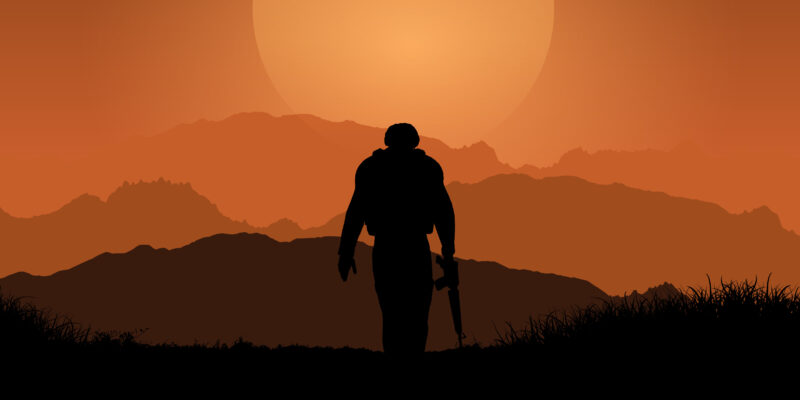The image is a horizontally oriented, digitally created graphic that combines multiple layers to create depth and atmosphere. Dominated by shades of orange and brown, the backdrop features a large, setting yellow sun partially obscured by clouds, casting an array of orange hues across the sky. In front of the sun, the silhouette of distant mountains fades from tan to gray and finally into black as they edge closer to the foreground. 

In the immediate foreground, there is a dark, detailed silhouette of a man, possibly a soldier. He is depicted standing on a hill, adorned with a helmet, body armor, and a backpack. The figure holds an assault rifle in his left hand, and his stance suggests he may be contemplating something or looking down. The overall scene, with its layering, gives an impression of the soldier walking into the sunset, creating a dramatic and somber mood.